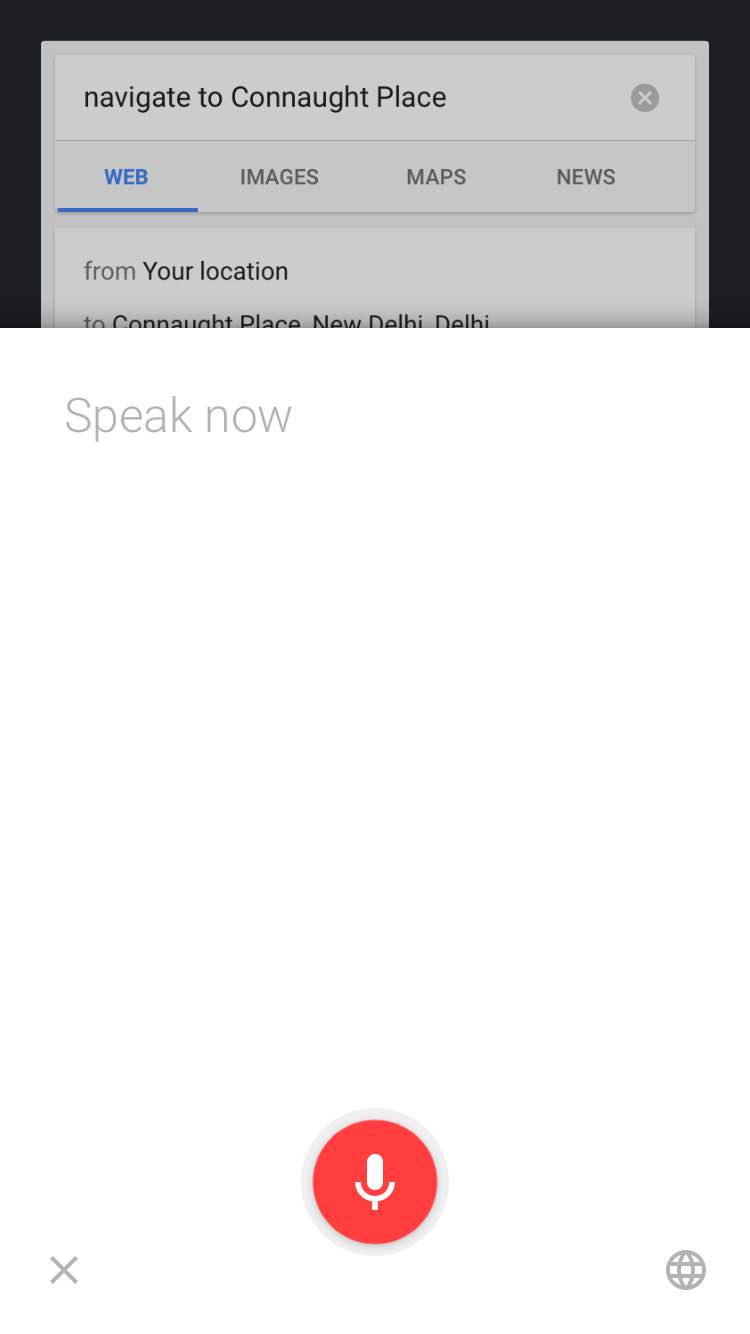This image is a screenshot of a smartphone where the voice input function has been activated for an artificial intelligence assistant. In the foreground, three-quarters of the screen is dominated by a white overlay with the prompt "speak now," indicating that the device is ready to transcribe spoken words. At the bottom of this overlay, a prominent red microphone button is visible, which the user must press to initiate voice input. Adjacent to this are two smaller gray buttons: an "X" for canceling the operation and a globe icon for changing the language settings.

In the background, partially obscured by the voice input overlay, the underlying page appears to be a Google search results page. The user had previously entered a search query for "navigate to Connaught Place," suggesting they were looking for directions. It seems that the initial text input method was either unsuccessful or unsatisfactory, prompting the user to switch to the voice input feature to achieve better results.